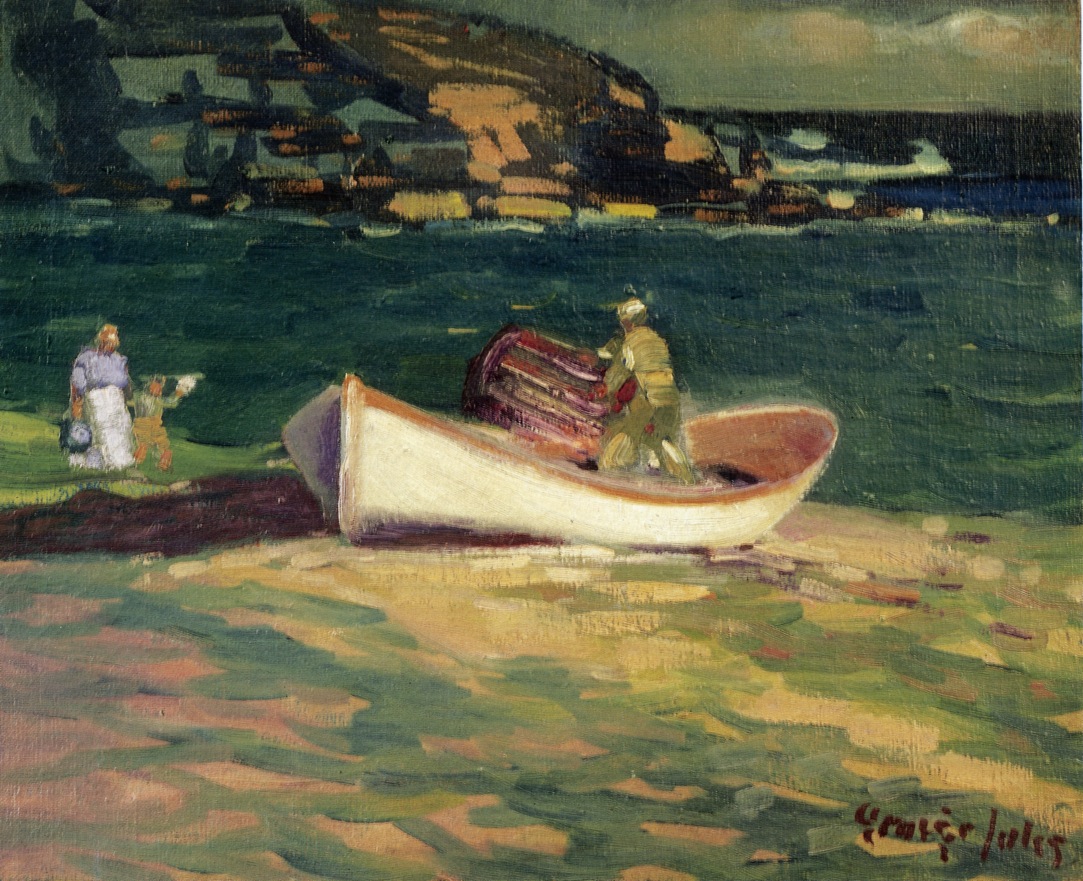This oil painting, depicted in a horizontal rectangular format, illustrates a dynamic scene with rich details and a somber mood. At the center sits a man aboard a modest, white rowboat with a light brown interior. The man, clad in an olive green vest, matching pants, and a cap, appears to be either preparing to cast or handling a fishing net or crate, suggesting he might be a fisherman departing for the sea. The boat rests at the edge of the shore, on a patch of beige, yellowish sand accented with dark brown dirt and surrounded by textured, foamy water.

On the left side of the painting, a woman in a white skirt stands with a child in tan pants who appears to be waving, possibly bidding farewell to the man in the boat. The scene is further enriched by the contrasting colors of the water: light orange and yellow hues near the shore transitioning to a dark green in the depths.

In the background, rocky hills adorned with homes and buildings rise on the left, while the right side opens to a dark, turbulent sea under a sky filled with ominous clouds. The artist’s red or dark red signature and the year of completion are faintly visible in the bottom right corner, adding an authentic touch to the emotive coastal scene.